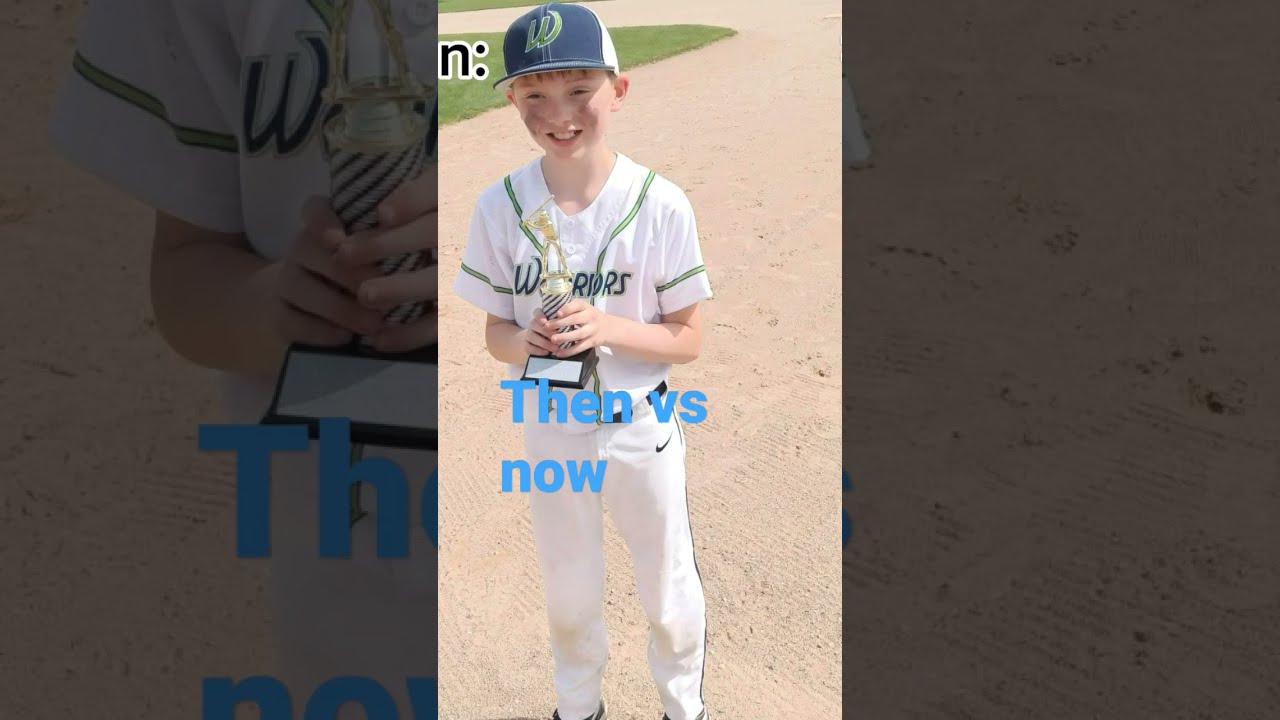The image depicts a fair-skinned, young Caucasian boy, likely between 8 to 12 years old, standing on a baseball field with sandy running paths and a strip of grass. He is dressed in a white Little League baseball uniform adorned with green pinstripes on the shoulders and elbows, as well as a blue and white cap featuring a green capital "W." Across the front of his jersey, the word "Warriors" is written in green. The boy is smiling, appearing happy, and his cheeks have some dirt smudges, suggesting he has been playing. He holds a gold trophy in his hands, and over the image, blue text reads "Then vs. Now." The central photograph of the boy has been placed atop an enlarged, darker copy of the same image, with the left third showing an up-close, darkened view of his arm holding the trophy, and the right third displaying a magnified, grayscale view of the sandy ground.